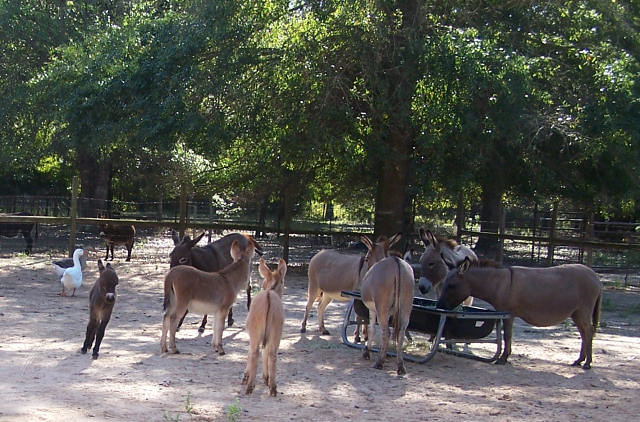This detailed outdoor photograph depicts a serene farm scene featuring eight donkeys and a solitary white duck amidst lush greenery and sturdy fencing. The donkeys, varying from dark gray to light gray, are stationed on light brown, sandy soil beneath a canopy of trees with abundant green leaves. They appear well-fed, with four donkeys eagerly feeding from a robust trough featuring a metal piping frame and a black bowl, while the remaining four donkeys stand leisurely, unhurried and content. The wooden posts with mesh or metallic fencing effectively enclose the area, suggesting a safe and animal-friendly environment. Notably, a baby donkey is positioned slightly in front of the duck, both facing the camera. This idyllic farm or petting zoo scene is captured on a bright, sunny day, accentuating the peaceful coexistence of the animals.